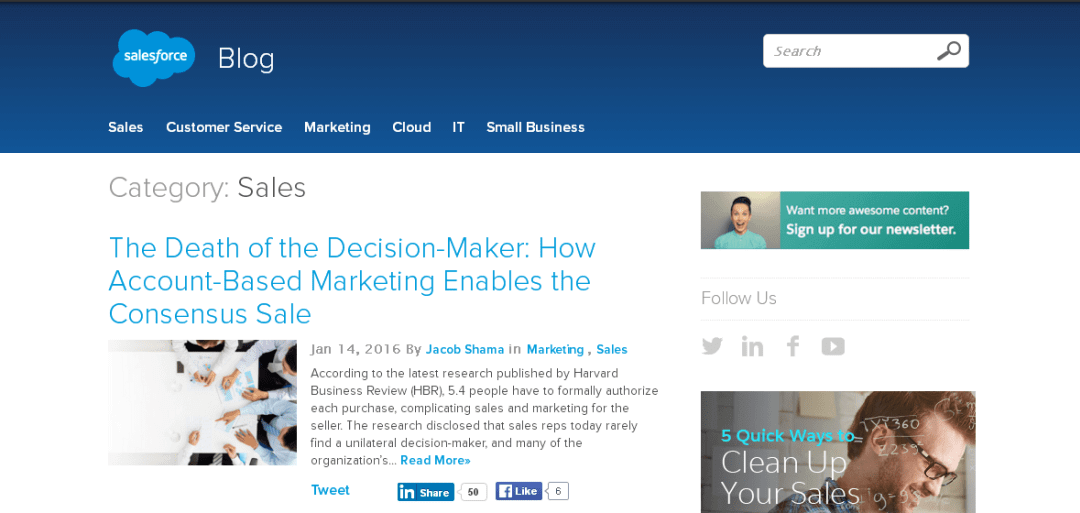The image is a screenshot of a Salesforce blog web page. Dominantly featuring a blue background at the top, the page is well-organized with a variety of navigational and functional elements. In the upper right corner, there is a search box designed for easy access. The top section of the screen lists several categories including Sales, Customer Service, Marketing, Cloud, IT, and Small Business, each likely leading to different sections within the site.

The Salesforce logo is prominently placed at the top left corner. It is designed as a puffy blue cloud with the word "Salesforce" inscribed in white, and the term "Blog" is seen nearby. Below this header, there is a category marker indicating 'Sales'. 

In the central section of the page, there is a featured blog post titled "The Death of the Decision Maker: How Account-Based Marketing Enables the Consensus Sale." This post is attributed to Jacob Shama under the categories Marketing and Sales, dated January 14th, 2016. 

Further down, social media buttons are visible, providing options to follow Salesforce on Twitter X, Instagram, Facebook, and YouTube, enhancing the page's social connectivity.

In the bottom right corner, an additional promotional graphic or advertisement highlights "Five Quick Ways to Clean Up Your Sales," offering a quick tip resource for sales improvement. Overall, the screenshot captures a well-structured Salesforce blog page focused on delivering insightful content related to sales and marketing.